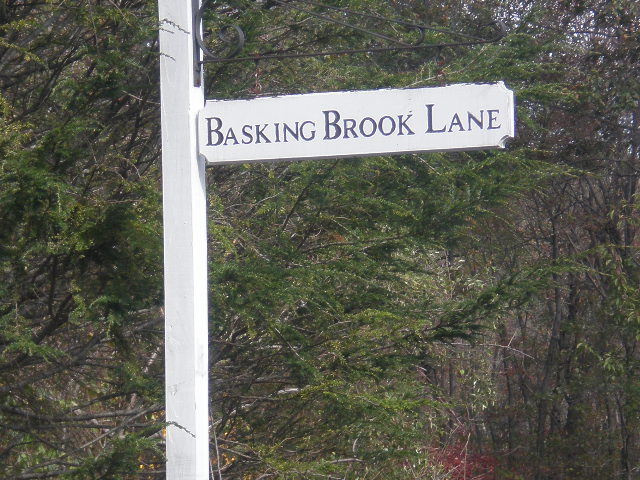The photograph captures a close-up shot of a rustic wooden signpost featuring a wrought iron hanger. Suspended from the iron hanger is a clean, white-painted sign with the bold black lettering "Basking Brook Lane." The signpost stands vertically, its weathered wooden texture suggesting it has been a fixture for some time. Background elements add a visual contrast to the simplicity of the sign; a dense, verdant mix of small trees and possibly some bushes forms a lush, green backdrop, enhancing the rustic charm and tranquil atmosphere of the scene. The image is taken from such proximity that it encloses just a section of the sign, withholding any view of the ground or sky and thus making it difficult to gauge the signpost's full height. The photograph's tight framing places emphasis on the sign's details and the natural elements immediately surrounding it, inviting curiosity about the secluded path it marks.